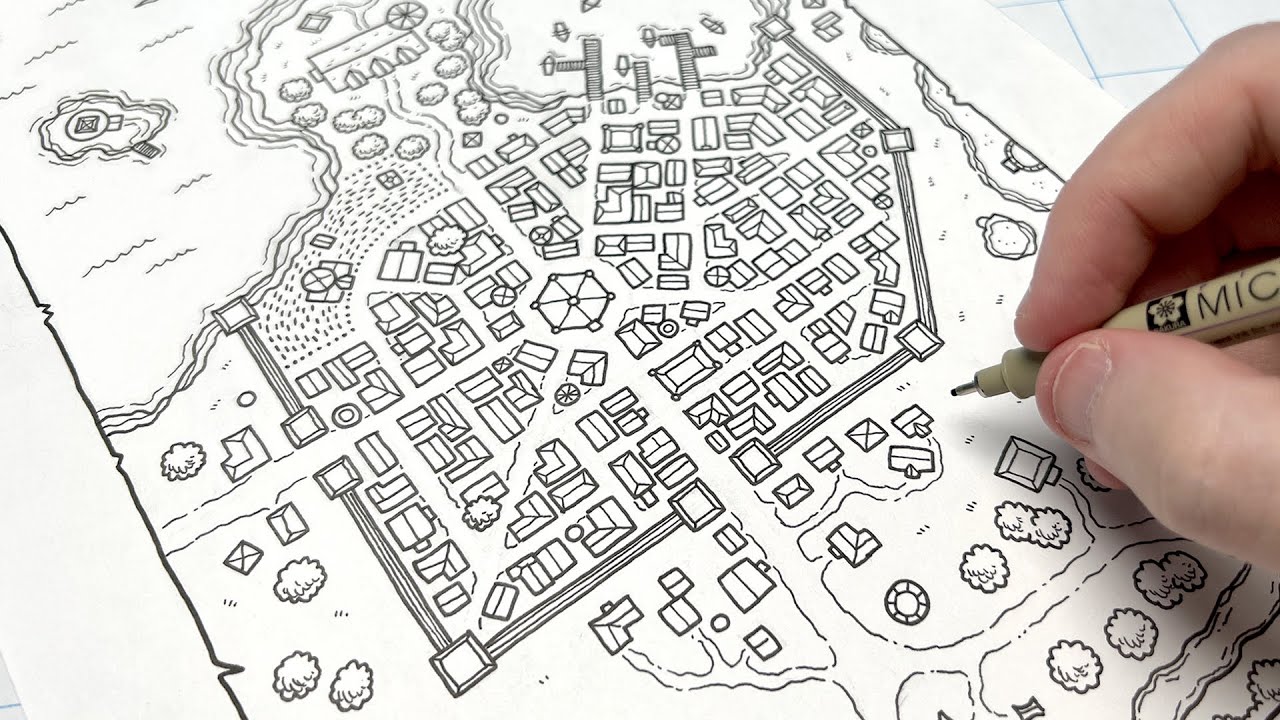This detailed photograph captures a white hand with very short fingernails, skillfully holding a light gray Micron pen marked with the letters "M-I-C" and a small black square featuring a flower design. Subtly positioned on the right side of the image, the pen's dull point touches down on a piece of paper that appears to be either a piece of wood or a gridded white sheet with faint blue lines. The main focus of the sketch is an intricate, black-and-white floor plan or overhead map of a town. Central to the drawing is a larger area, potentially representing a circus tent or a cul-de-sac, with roads branching out in various directions. To add depth to the scene, there are detailed illustrations of trees, a river denoted by a squiggly line at the top, and a walled-in section that encloses smaller houses, bushes, and other buildings. The top right section of the map reveals a dock area with piers and tiny sailboats, while an ocean segment with an island lies further left. Additionally, there's a notable structure resembling a church nestled between these two areas. The outer edge of the map is framed by a black line with angular notches, completing the intricately detailed piece.